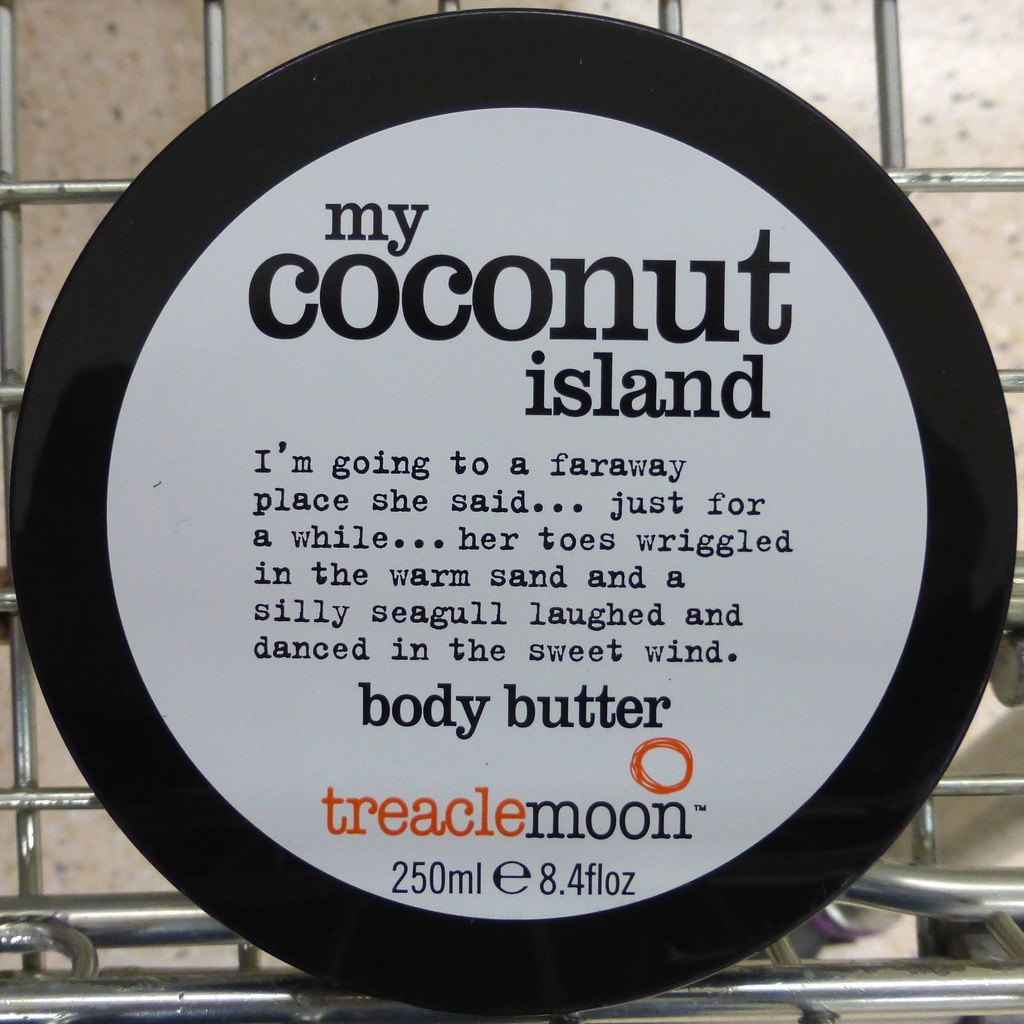The photograph, taken indoors, captures a sign nestled inside a metal shopping cart, with the cart's characteristic metal bars clearly visible. The sign, seemingly the lid of a jar, is oval-shaped with a black border encasing a white background. Predominantly, the text on the sign is black, accented with a touch of orange. At the center, the bold black lettering reads "My Coconut Island," followed by a whimsical narrative: "I'm going to a faraway place, she said... just for a while... Her toes wiggled in the warm sand, and a silly seagull laughed and danced in the sweet wind." Beneath this, the text "Body Butter" is displayed in black, and in orange, the word "Treacle," followed by "Moon" in black. The sign, likely the top of a body butter jar, details the product's quantity as 250 milliliters (8.4 fluid ounces). The overall setting and composition suggest it is an advertisement for Coconut Island Body Butter by Treacle Moon.